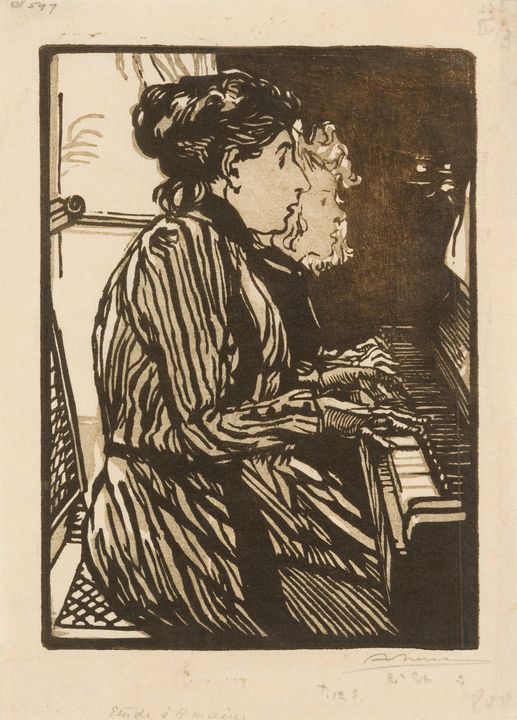The image is a detailed black and white artwork depicting an older woman and a younger lady seated side by side at a piano, likely from a nostalgic era reminiscent of the 1800s. The older woman, with dark hair pulled back into a loose bun, is dressed in a high-collared, black and white striped dress with long sleeves extending to the floor. Beside her on the same bench is a younger lady with short, curly blonde hair, dressed in a dark dress. Both have their hands poised over the piano keys, possibly engaged in a piano lesson or playing together. The piano extends slightly into the right side of the image, showcasing a layout with white keys in the front and black keys at the back. In the background, a black wall dominates two-thirds of the image, broken by a window in the top left corner allowing a sliver of light to filter through. The image captures a moment of quiet concentration and shared musical endeavor between the two figures.